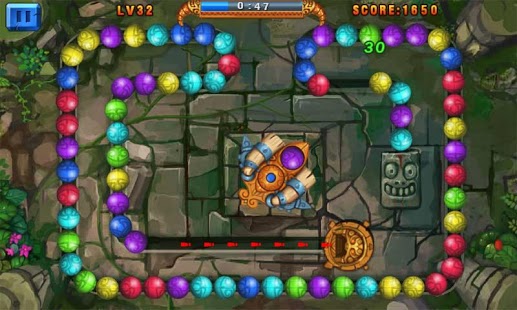This image is a detailed screenshot from a mobile app game with a timed objective. Set against an ancient jungle-themed stone background with various vegetation, including purple flowers and bushes, the game features a winding pathway formed by numerous colored balls or beads arranged in a seemingly random order: purple, blue, yellow, green, and so on. These balls appear to be emitted from a gold-like, face-shaped apparatus on its side, spitting out red-tailed dots that likely represent each new ball. On the right end of the pathway, there is a large rectangle sporting a goofy face, serving as a target for the balls. 

In the middle of the scene, a special apparatus containing a jewel is prominently displayed. Positioned at the top center, a timer indicates there are 47 seconds left, alongside a filled progress bar. Further, an orange font signifies that the player is on Level 32, displayed as "LV32," with a current score of 1650 points. In the top right corner, a green number 30 suggests recent points added to the score. The background is enriched with stone structures, contributing to the game's immersive ancient setting.